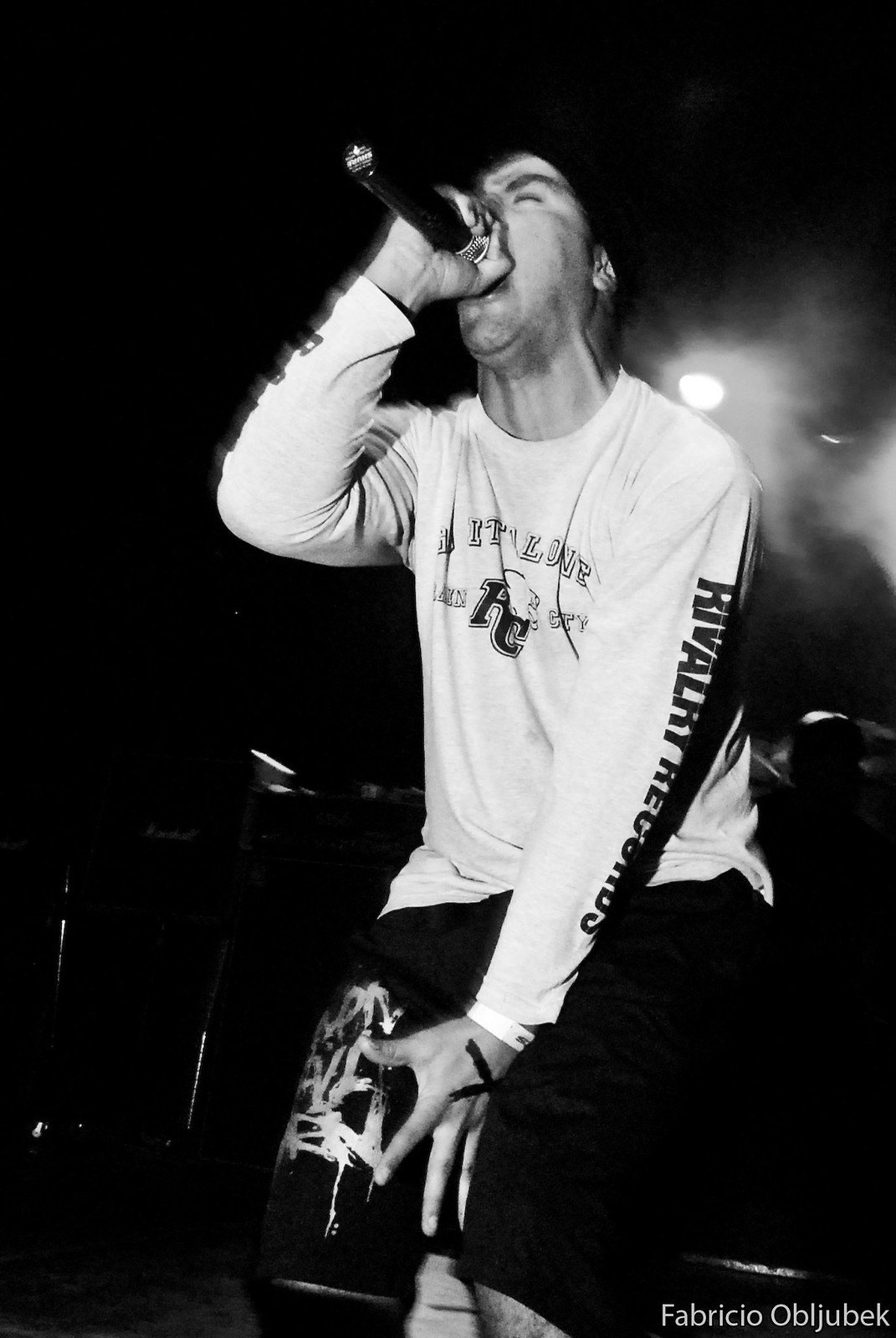The black-and-white photograph captures an emotionally charged moment at a concert. A man, possibly in his thirties, is depicted screaming emphatically into a microphone that he grips tightly with his right hand. His intense emotion is evident in his partially closed eyes and the forceful posture of his mouth against the mic. He is wearing a white long-sleeve shirt and black pants, with some indiscernible white pattern or possibly spray-painted words on his left leg. The pants appear to be shorts, revealing his knee. His left hand is dramatically reaching across his body, grasping his left leg. The background is dark, making details hard to discern, but a single stage light shines behind him, casting light through wisps of smoke or mist. Over his left shoulder, a hint of a drum set is faintly visible, catching some light. The bottom right of the image features white text reading "Fabrizio Oblige Beck." The raw energy and passion of a heavy rock or metal performance are palpable in this powerful image.